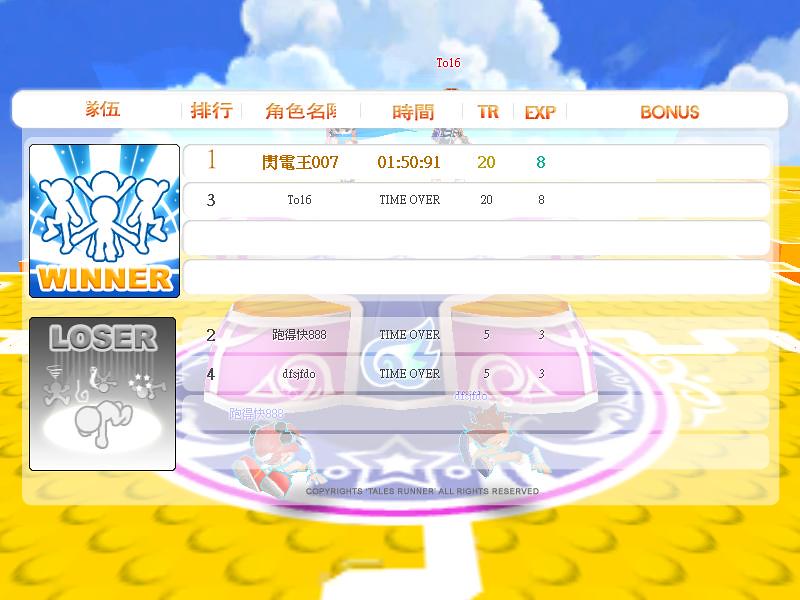The image is a computer-animated screenshot from a video game, likely "Tails Runner," as indicated by the copyright notice at the bottom. The top of the image features a cartoony, blue sky with scattered white clouds. Below the sky is a yellow background adorned with small white lines, overlaid by three white-bordered sections.

In the upper section, Mandarin characters are present alongside abbreviations "TR," "EXP," and "bonus." Below this, there is a square labeled "Winner," showcasing four jubilant white figures against a blue background with white lines. The figures appear to be jumping with arms spread out. To the right, numbers and additional Mandarin characters appear, including "1," "007," "01:50:91," "20," and "8."

The middle section features a different scoring segment marked by "3," "TO16," and "time over 28." On the bottom left, the word "Loser" is displayed next to a group of four characters who look unhappy, some bent over with stars over their heads or a tornado, set against a gray and white background. Further annotations include "2," Mandarin characters, "888," and "time over 5:3," followed by "4," and "DFSJFDO."

At the very bottom of the image, a footer states: "Copyrights, Tails Runner, All rights reserved."